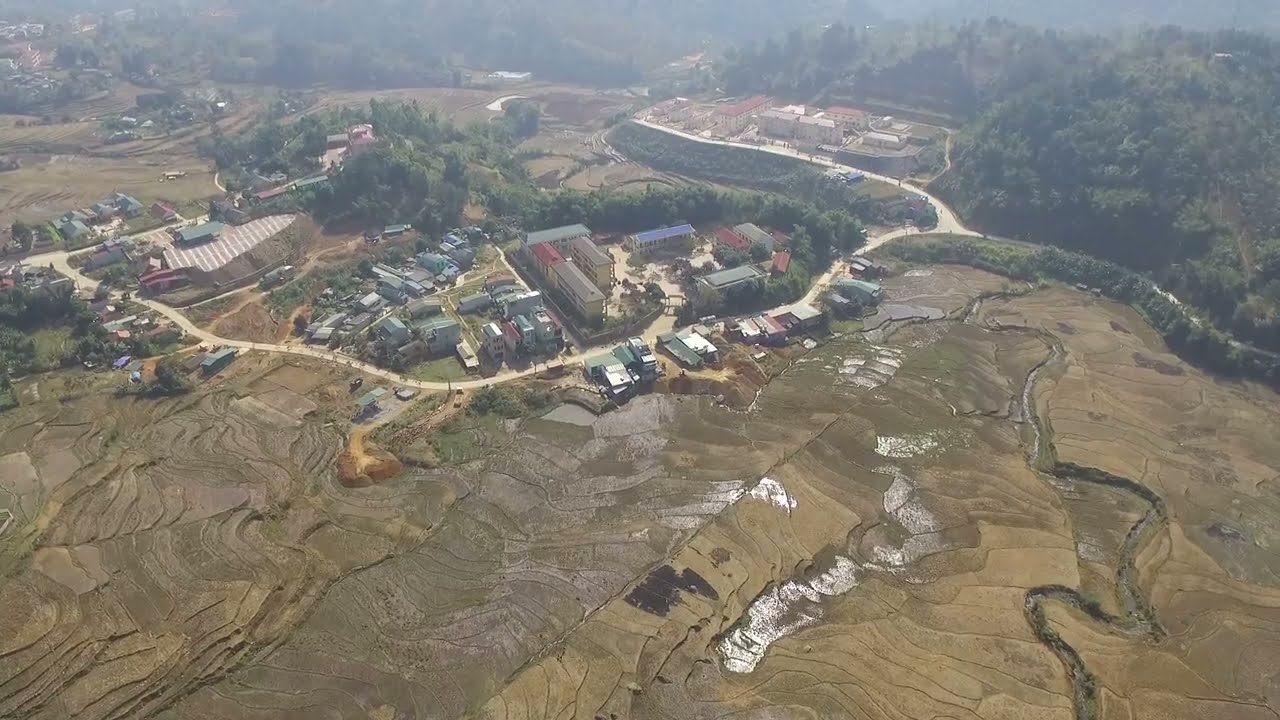This aerial photograph captures a detailed overhead shot of a landscape during the day. Central to the image is a dry, snake-like stream bed meandering from the bottom center toward the top center, surrounded by brown, swirled, and contoured ground indicative of past water runoff. The landscape is primarily flat and dry, possibly consisting of dirt or dead fields, with misty or foggy elements softening the distant background. On the right and left sides of the image, glimpses of a small town emerge, with clusters of buildings and homes. Roads interweave through the scene, extending from the left side, traversing towards the top, and then connecting to the right. Additional details include vehicles visible on these roads and patches of greenery and small ponds scattered throughout. The far background reveals a more lush and forested area, providing a stark contrast to the barren foreground. The image does not include any people, animals, or the sky, focusing solely on the terrestrial landscape and its features.